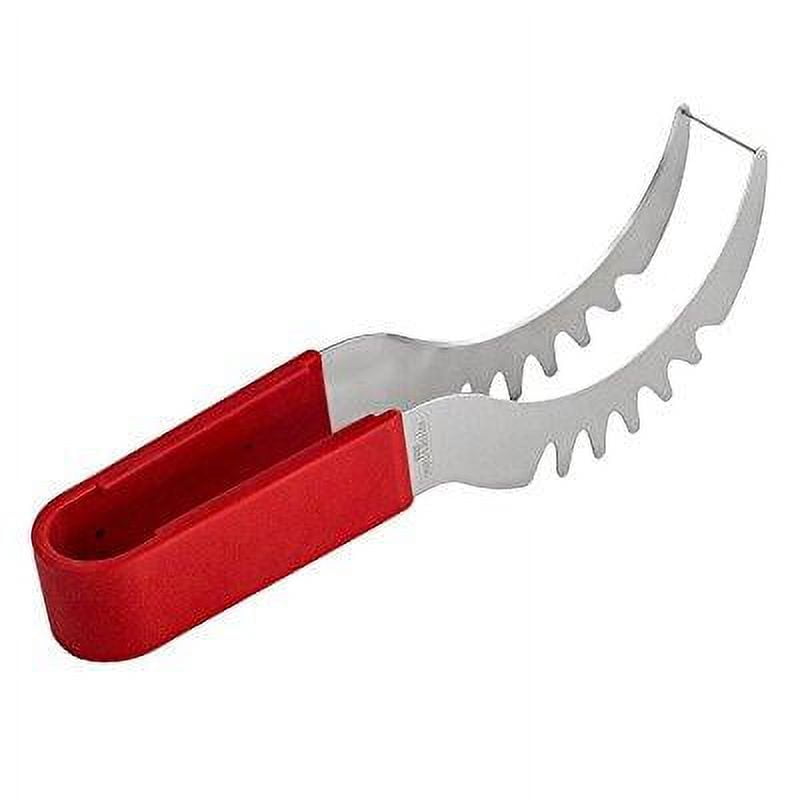In this image, we see a specialized tool with a distinctive red, handle-shaped bottom part, reminiscent of a bar magnet that is hollow and bends upwards in the middle. The overall structure is blurred, and the background is a plain white, giving the impression that this might be an advertisement focusing solely on the tool. The handle transitions into a silver-colored section featuring sharp, knife-like projections, forming an array of five teeth-like blades designed for gripping. These blades, which are mirrored on both sides of the tool, are connected at their tips by a very thin black rod. Additionally, there's faint, unclear text on the side of the handle. The tool appears to be designed for precision tasks, with its angled and curved shape suggesting it could fit into small or tight spaces.